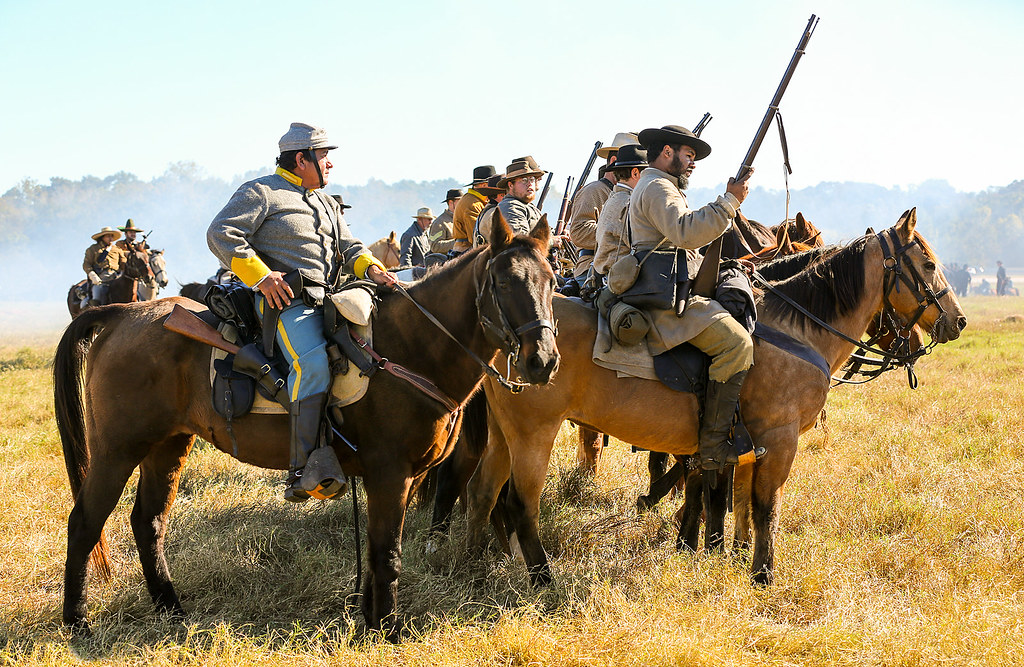This image captures a highly detailed scene of what appears to be a Civil War reenactment set in a expansive grassy field. The foreground features numerous men on horseback lined up in two distinct rows, with the majority of them clad in heavy gray wool uniforms indicative of Civil War era attire. These uniforms include flat hats with rims, and several of the men are wielding large, musket-like rifles, with one notable soldier in the front row perching his musket on his right thigh. A light brown horse stands among the group, facing the camera and drawing attention with its direct gaze.

One of the prominent figures stands out due to his distinctively bright blue pants adorned with a yellow stripe, contrasting against his gray wool jacket. This individual also sports a hat with a chin strap and strikes a confident pose with his left hand gripping the rein and his right hand resting on his hip. The reenactors on horseback appear to be at attention, with their mounts' legs hanging straight into the short, yellow-green grass of the field. 

The background reveals misty, out-of-focus mountains and a forest, under a blue and white sky. Additional figures on horseback can be seen riding in from the left, while others stand dispersed towards the far right. The composition and clarity of the photo suggest it was taken recently, capturing the reenactors amidst a moment frozen in time.